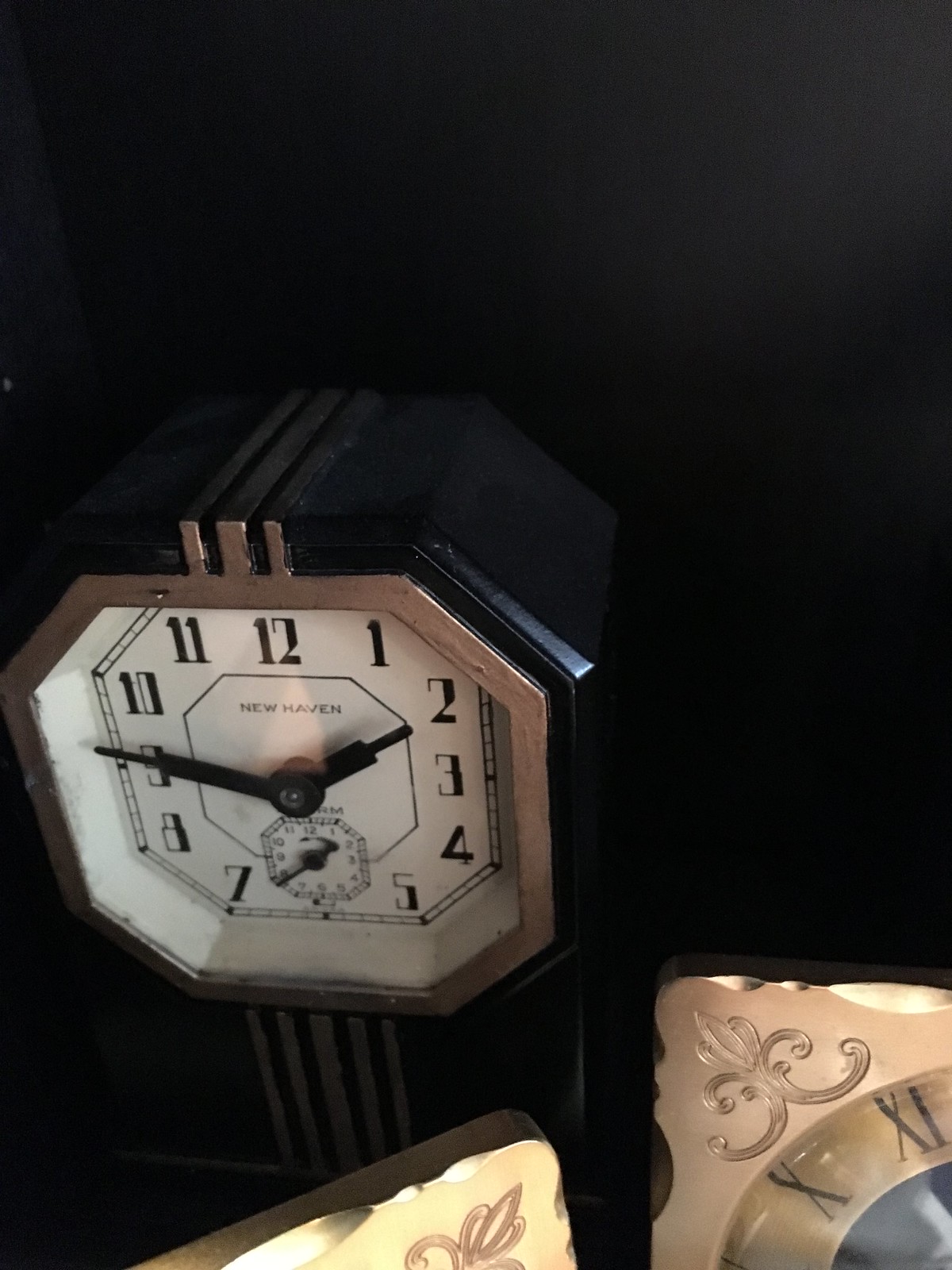In this very dark image, the primary focus is on an elegantly designed clock with a black and gold color scheme. The main clock prominently displays the name "New Haven" and features a white-faced hexagon at its center, bordered by gold. Inside this hexagonal section, the clock boasts Art Deco-style numerals and includes a smaller clock face dedicated to seconds. This smaller face is intricately detailed within the larger design. Positioned on a reflective surface, the clock’s gold and black elements are mirrored subtly below it. In the bottom right corner, part of another clock is visible, highlighted by Roman numerals X (10) and XI (11) on a gold background. Additionally, the tip of yet another clock can be seen entering the frame from the bottom left, contributing to the overall composition that suggests a collection of timepieces displayed together. The time on the primary clock reads exactly two forty-six.